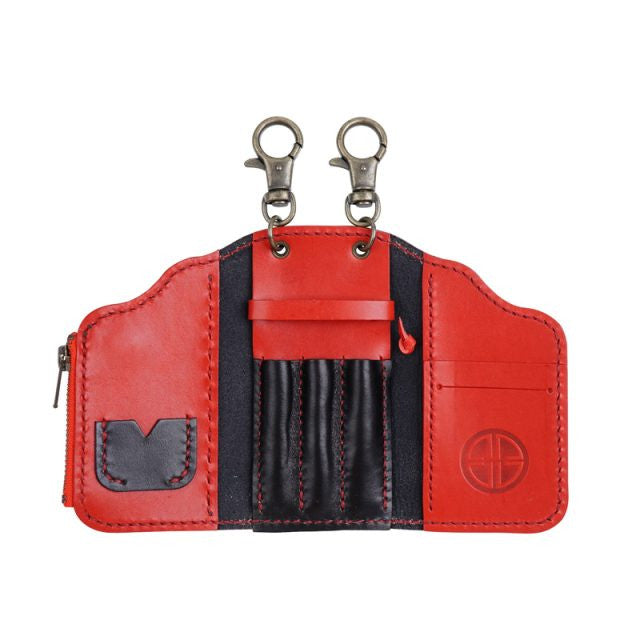This image showcases an up-close view of a multi-functional red leather wallet with a unique design, likely serving as both a wallet and a keychain holder. The wallet features a distinctive wide rectangular shape with a scalloped top edge, which is taller in the middle and tapers down towards the sides. The dominant red leather exterior is complemented by intricate red stitching.

On the left side, there is a visible zipper running along the edge. Inside, a black leather U-shaped pocket is sewn onto the red background with red thread, potentially useful for small items or coins. Adjacent to this pocket is a black leather section that offers an additional compartment, suitable for cash or cards.

In the central part of the wallet, there is a black background with a small red square at the top. Two silver clips, resembling round grommets, protrude from this section, designed to attach to belt buckles or other items. Below the clips is a black section segmented into three pockets, presumably for holding pens or similar objects.

The right side of the wallet features a red panel with a slot, ideal for storing credit cards or identification. The panel also displays a circular logo, adding a touch of branding to the piece.

Overall, this detailed red leather wallet combines functionality with aesthetic appeal, offering specialized compartments and attachments for versatile use.